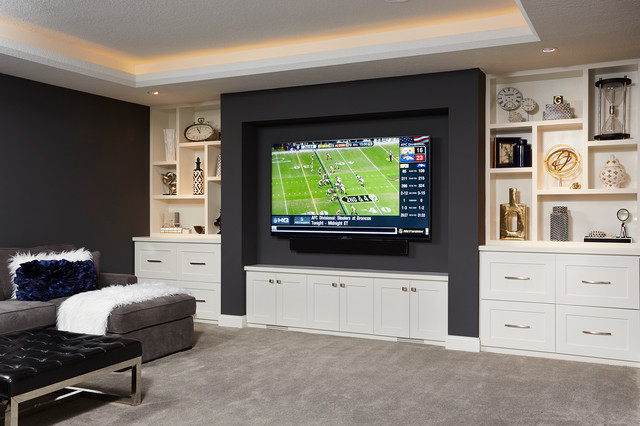This detailed photograph showcases a meticulously designed modern living room. Dominating the center is a large flat-screen TV, approximately 70 inches in size, broadcasting a football game. The TV is mounted within a dark gray inset wall that contrasts sharply with the surrounding white storage units. These units feature built-in shelves adorned with an array of artistic objects, such as clocks, glasses, sculptures, vases, and an empty hourglass. Below the TV, white cabinets and drawer sets with silver handles offer additional storage, enhancing the room's modern aesthetic.

On the left side of the image, part of a comfortable seating area is visible. A dark gray sofa is covered with a fluffy white blanket and adorned with plush blue and white pillows. A black leather ottoman with metal trimming sits nearby, complementing the soft light gray carpeting that spans the floor.

The room is further illuminated by recessed lighting set into an inset white ceiling, casting a bright and inviting glow over the entire space. This clean and organized living room offers a striking mix of dark and light tones, showcasing both function and style.